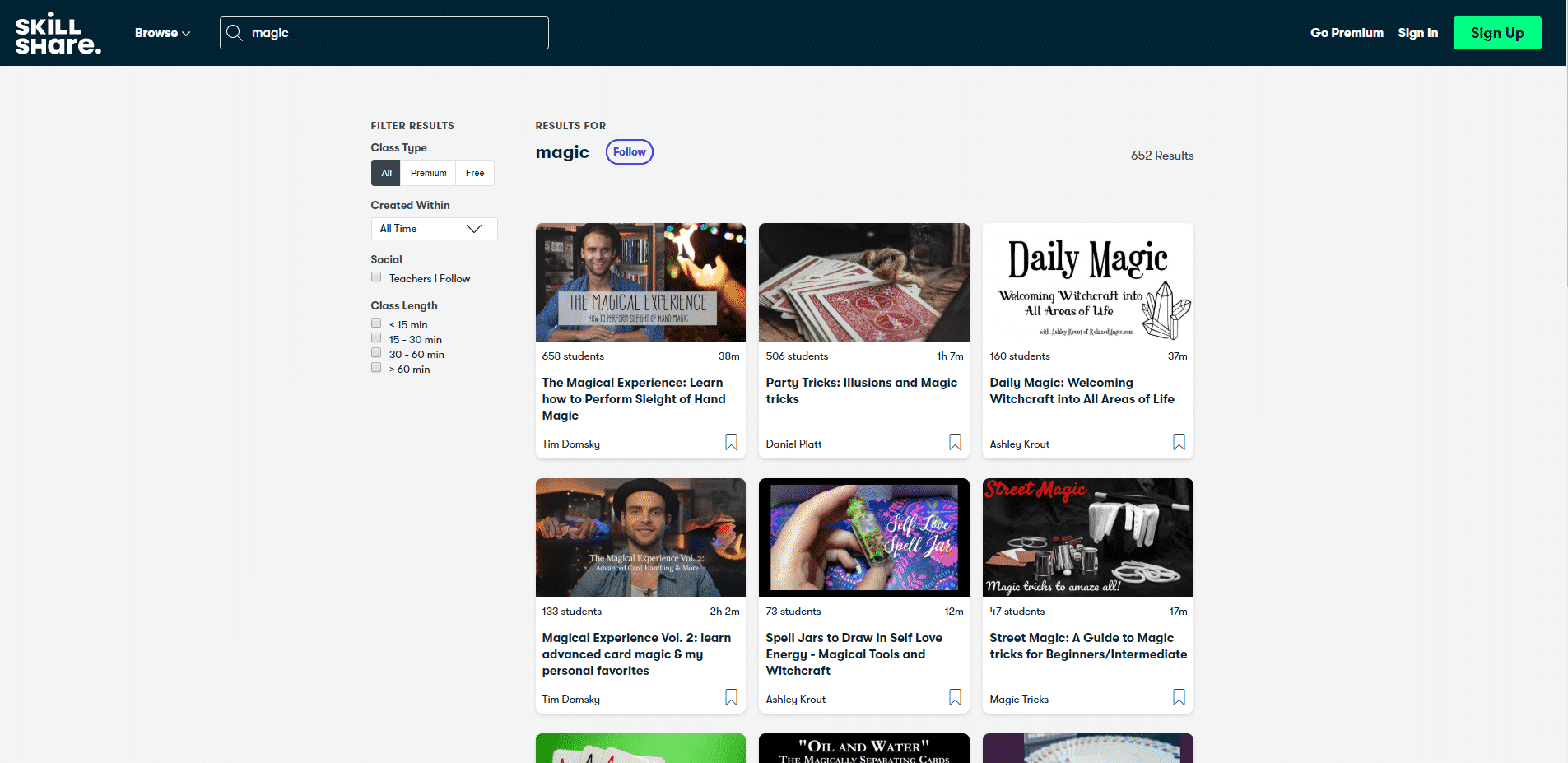The rectangular image features a detailed interface of the Skillshare website. At the top of the image, there's a black header bar displaying "Skillshare" in white text. Below this, on the left side, is a navigation section starting with the word "Browse" accompanied by a drop-down arrow. Adjacent to it is a search box with a magnifying glass icon, populated with the text "magic." 

To the right of the search box, the options "On Premium" and "Sign In" are displayed. Further right, there's a prominent green button with the text "Sign Up" written in black. 

The background color below the header transitions to light gray, forming the main body of the interface. On the left, there's a vertical menu titled "Filter Results," with a section labeled "Class Type." The option "All" is selected by default, followed by additional selections for "Premium" and "Free" classes. Below, there's a drop-down menu for "Created," although the rest of the menu options are difficult to decipher due to their small size.

Towards the center, moving right, the title reads "Results for 'magic,'" accompanied by a purple-outlined box that features the word "Follow" in purple text. In the far-right column, a summary states there are "662 results."

The image showcases at least six search results for "magic," though some are partially readable. The first listed result is titled "The Magical Experience: Alecra – How to Perform Sleight of Hand Magic."